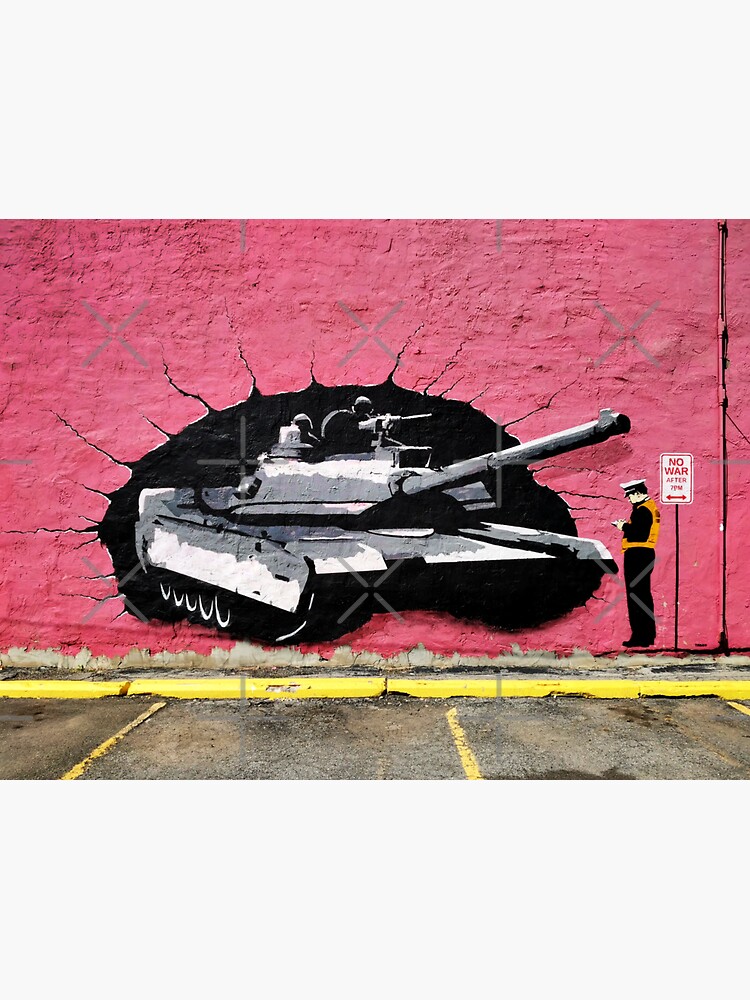This outdoor photo captures a mural painted on the side of a rough-looking, deep pink building. The mural artfully depicts a scene involving a street setting with a brown and tan painted pavement, featuring realistic yellow lines for parking spaces and a yellow curb. At the center of the mural, a military tank, rendered in gray, black, and white, emerges from a gaping black hole, its long front gun extending outward. Two military men are visible coming out from the hatch on top of the tank. To the right of the tank, a police officer dressed in a black shirt, black pants, and an orange vest stands, appearing to write a ticket. He sports a traditional cop cap and is shown from his left side. Behind the officer, a boldly painted sign reads "No War After 7 p.m." on a white background with red text. The mural creatively merges various elements, seamlessly integrating the painted street scene with the deep pink, roughly textured building facade.